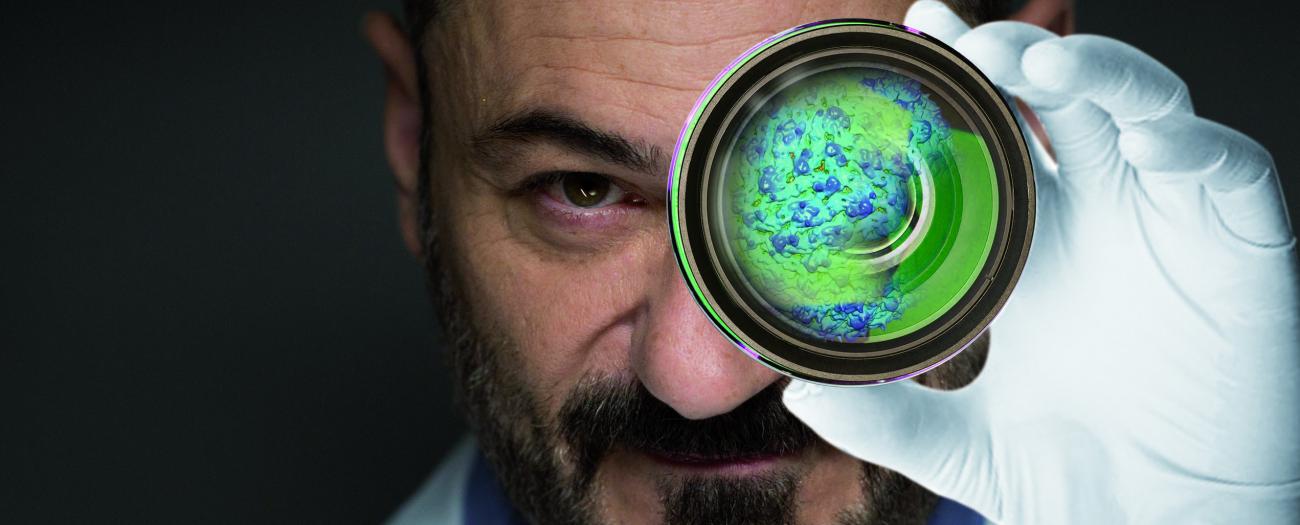In this image, a middle-aged Caucasian man with a neatly trimmed dark beard and mustache is staring directly at the viewer with his right eye while his left eye is obscured by a circular, glassy object that he holds up with his left hand, which is clad in a white glove. The object, resembling a petri dish or a lab specimen container, contains a vibrant green gel speckled with blue spots, which lends a neon glow to the scene. His forehead, marked with horizontal wrinkles, suggests a concentrated or curious expression as he examines the object. The stark black background emphasizes the dramatic, slightly surreal quality of the scene, which evokes the meticulous nature of scientific investigation. The man exudes a scientific aura, possibly hinting at a laboratory or research environment, and his eye visible through the dish appears to be dark brown or green, accentuating his intense scrutiny.